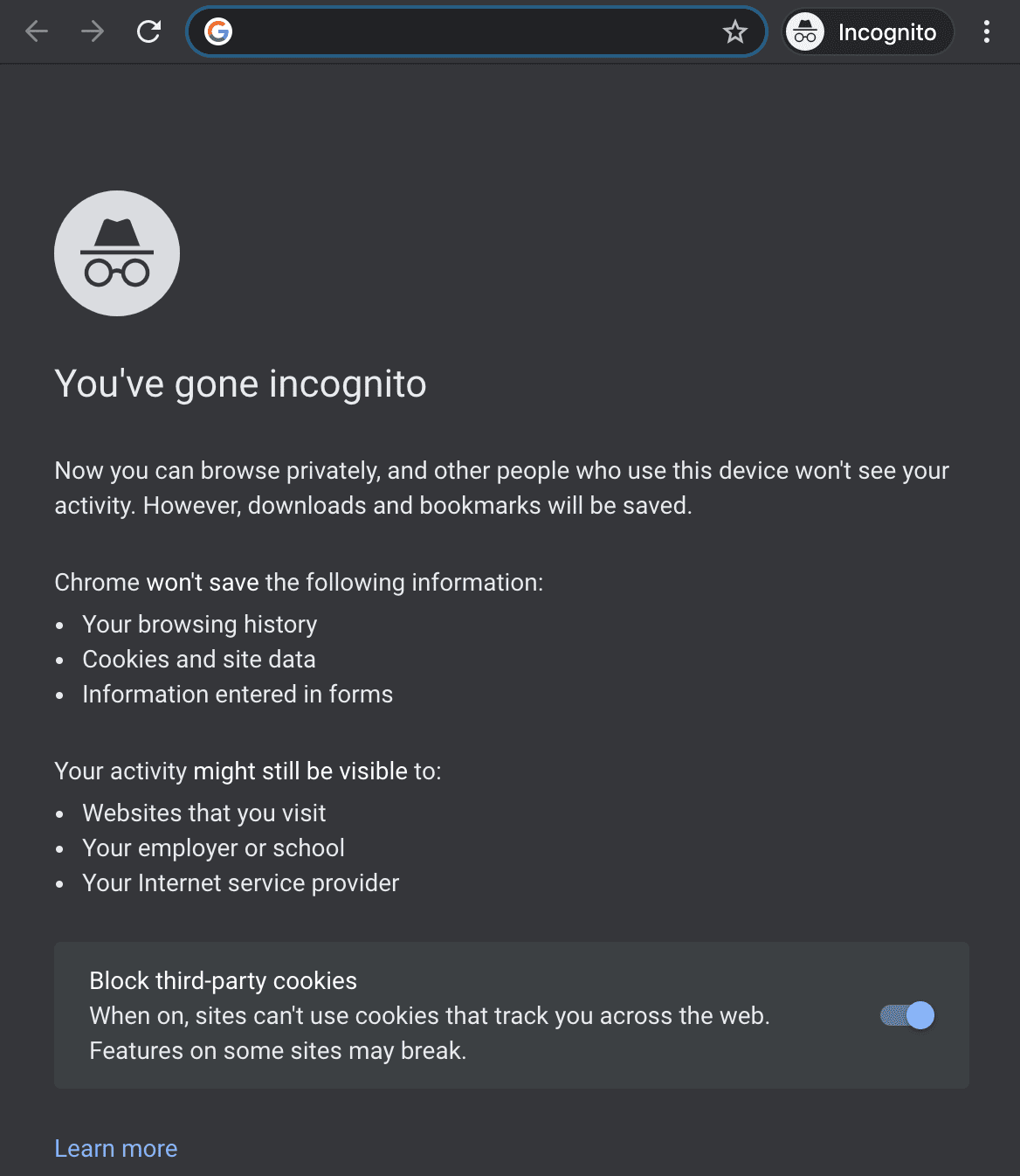In the image, the background is predominantly grey. In the top-left corner, there is a grey arrow pointing left and right, accompanied by a white refresh icon. Below this, there's a blue elongated circle featuring the Google logo on the right side, next to a white circle containing a grey star, all set against a black background.

Further down, there is a grey elongated rectangle displaying an icon of a fedora hat and glasses within a white circle, alongside the word "Incognito" in white font. To the right of this, three white vertical dots are aligned.

At the bottom of the image, another white circle features a black hat with a black rim and black glasses, set against a white background, with the text "You've gone incognito" beneath it in white font. Below this, a message reads: "Now you can browse privately, and other people who use this device won't see your activity. However, downloads and bookmarks will be saved."

The next section outlines what Chrome will not save: 
- Your browsing history
- Cookies and site data
- Information entered in forms

Following this, a cautionary note mentions that your activity might still be visible to:
- Websites you visit
- Your employer or school
- Your internet service provider

At the bottom, in a third box with white font, it states: "Block third-party cookies. When on, sites can’t use cookies to track you across the web. Features on some sites may break." To the right of this, there is a blue toggle switch (indicating it is turned on) with a grey outline circle on its left. The next line down features the phrase "Learn more" in blue font on the left side.